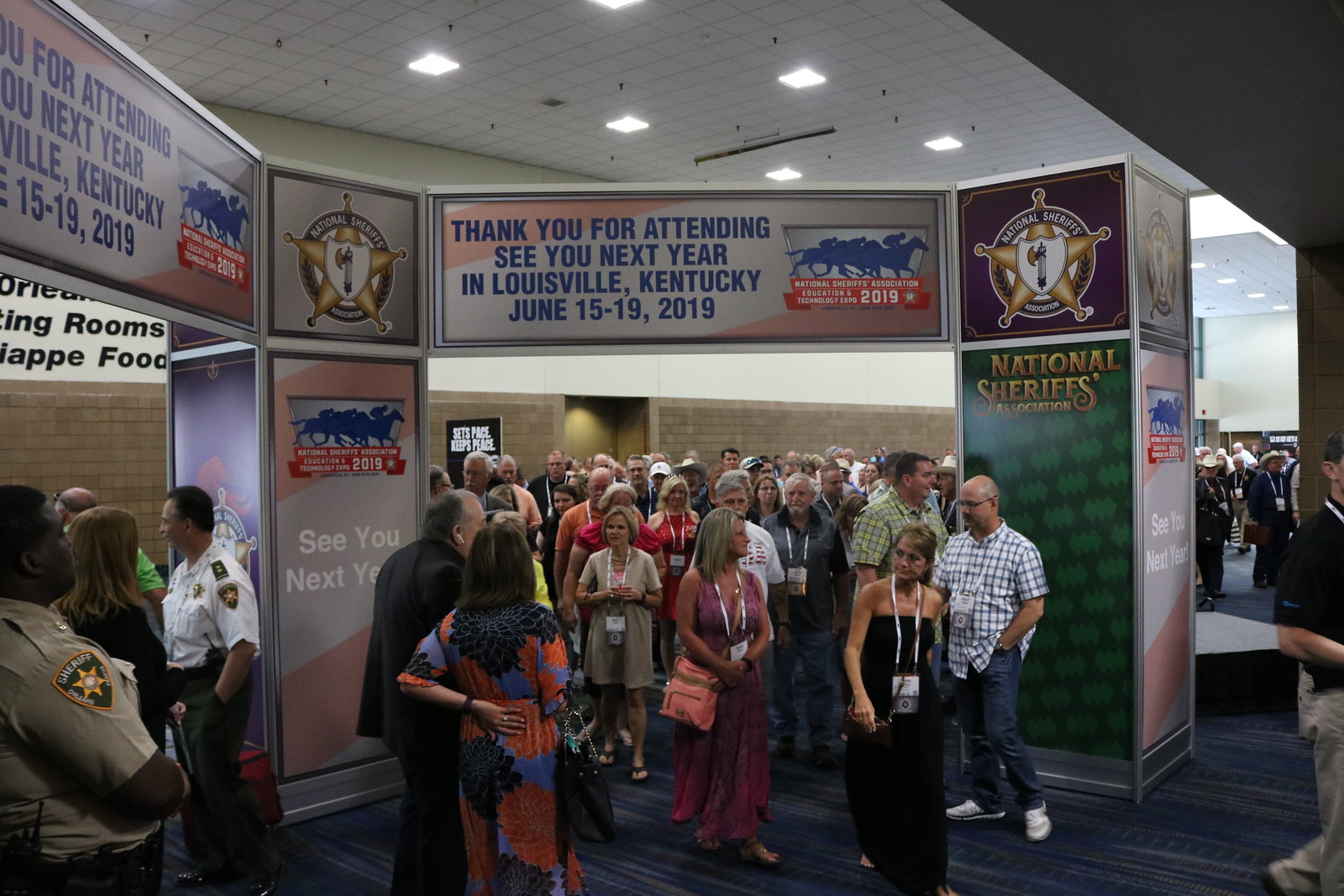This image captures a bustling indoor scene from a convention, with a large crowd of casually dressed individuals walking through the center. The floor is covered in carpet, and a variety of colors such as tan, black, white, green, orange, blue, purple, pink, gray, and brown are present throughout the image. Overhead, a distinct archway formed by two rectangular towers features several signs and advertisements. The right tower has a green section with gold lettering that reads "National Sheriffs Association," accompanied by a maroon section displaying a logo with a gold sheriff's star. The top portion of the archway, which connects both towers, has a black, red, and white striped background with blue text that says, "Thank you for attending. See you next year in Louisville, Kentucky, June 15th - 19th, 2019." This text is flanked by sheriff's star logos. To the left of the crowed scene are security guards, one in a white shirt and black pants. The setting appears to be a well-lit indoor space, indicating it is likely daytime.